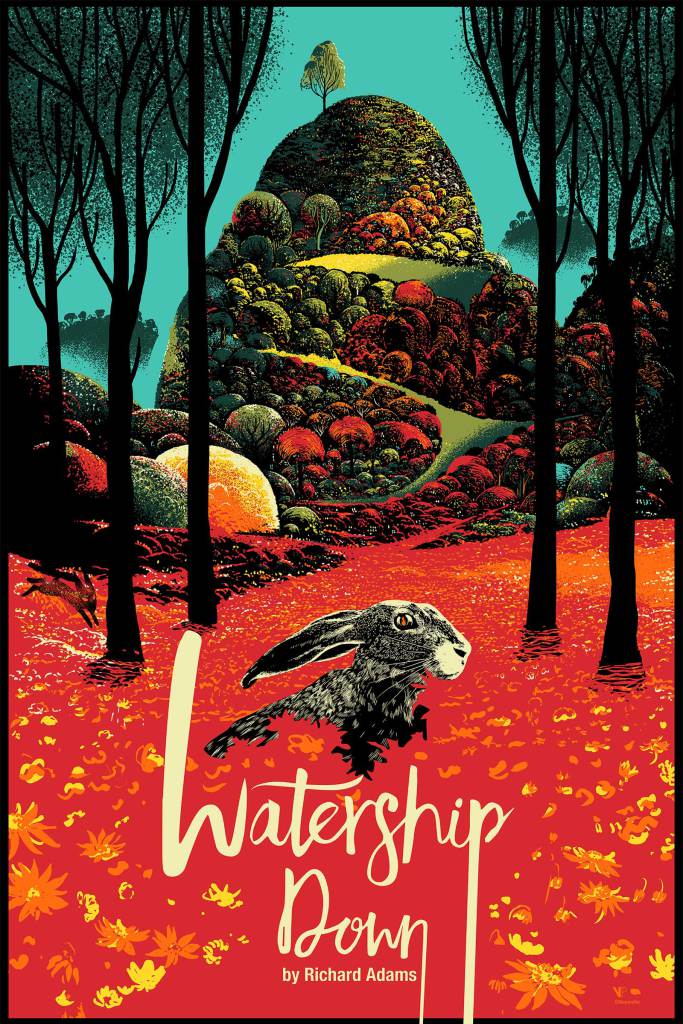The image is a detailed book cover poster for "Watership Down" by Richard Adams, with the title prominently displayed in cream-colored font at the bottom middle. The artwork features a whimsical, fantasy landscape dominated by a bright, aqua-blue sky at the top. Central to the composition is a steep hill adorned with a winding path and flanked by tall, slender trees topped with small, pinpoint leaves. The hill itself is dotted with small trees, while the path is lined with striking reddish rocks. A vibrant reddish-orange and yellow forest floor extends across the scene, giving way to a ground scattered with colorful shrubbery and plant life that appear round and bubble-like. Nestled among this vividly detailed wilderness is a gray bunny, depicted with its face turned to the right and ears laid back. This cohesive cover design captures both the richness of the natural setting and the ethereal quality of the story.